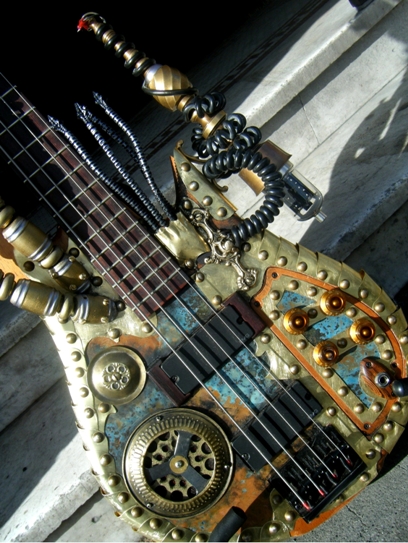The image depicts a highly customized and ornate four-string bass guitar, transformed into an intricate piece of art. The guitar's body and portion of the neck are lavishly adorned with a variety of embellishments, including brass and copper elements. The surface is decorated with button-like designs, small metal beads resembling the tops of screws, and elongated cylindrical objects. Additionally, it features gold medallions and blue metal pieces, enhancing its artistic appeal. The strings remain intact, and there are electrical components and what appears to be a device attached with an old telephone cord, possibly functioning as a microphone. The guitar is propped up against a set of white-colored stone steps, resting on a cement floor, with the neck angled upwards, leaning to the left.